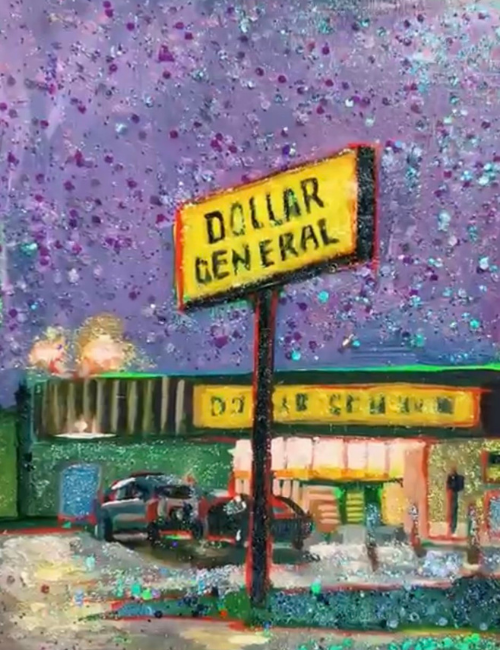This stylized painting of a Dollar General store features a striking background with a textured purple sky speckled with blue and white dots, giving an impression of raindrops. A prominent feature is the large yellow Dollar General sign at the top of a black and red pole, visible above the store. The sign itself is yellow with black lettering. Below, the store has green walls and a green roof, with a big glass front through which light shines, casting a warm glow. The scene also includes a standard parking lot with a black car and a silver car parked in front. Surrounding the store is a touch of greenery, adding a bit of natural color to the otherwise urban setting. The overall composition, with its rough brushstrokes and abstract elements, emphasizes the distinct figures and ambiance, making it evident that this is a Dollar General store despite the impressionistic style.